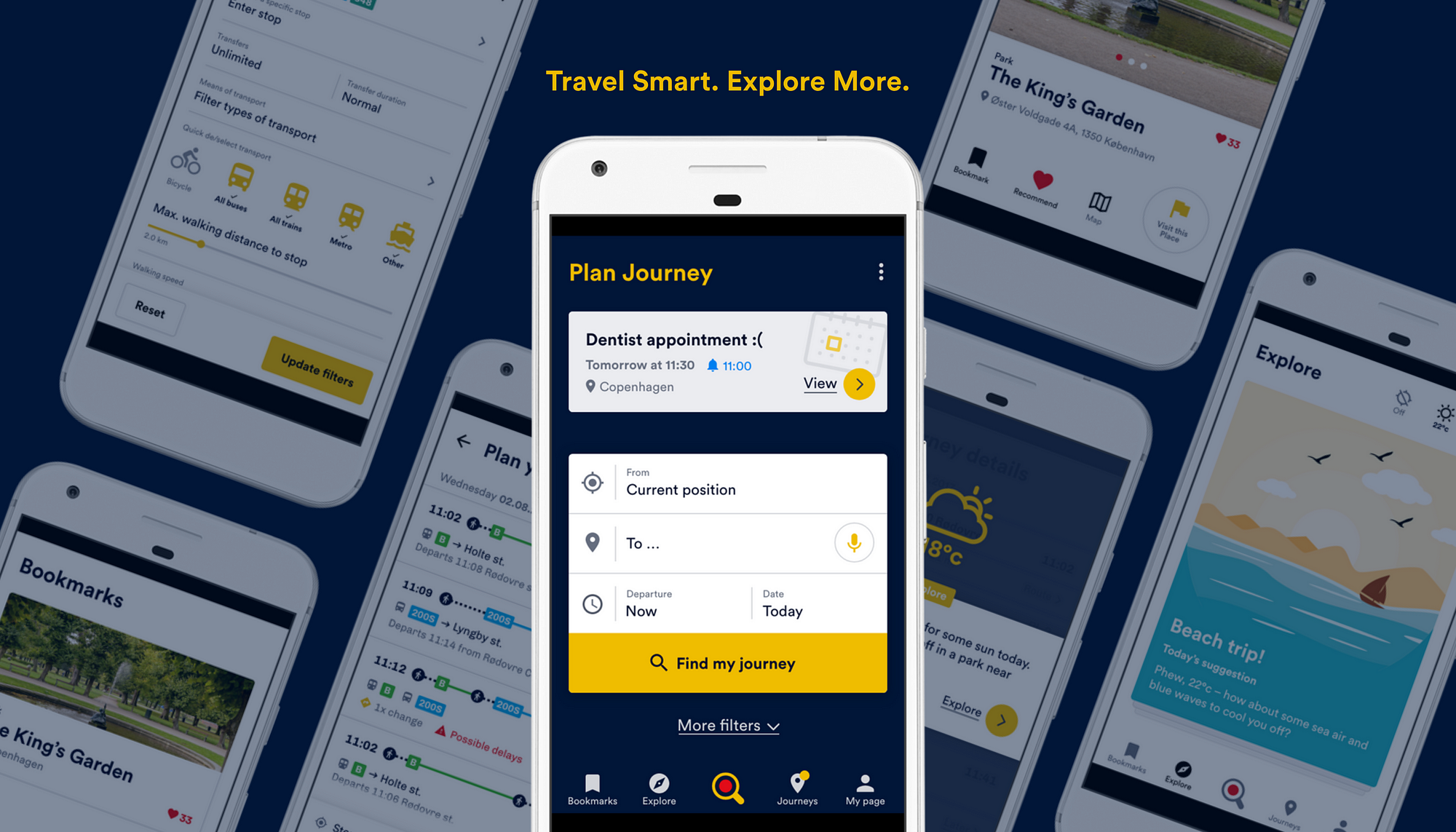This image features an advertisement, though it lacks any company branding. The header prominently displays the slogan "Travel Smart, Explore More." A smartphone occupies the central focus, showing a screen with various text entries, including a scheduled "Dentist Appointment Tomorrow at 11:30," and a planned journey to "Copenhagen from current position." The interface provides options like "Departure Now," "Day-to-Day," "Find My Journey," "More Filters," and buttons to "Take a Look at the Bookmarks," "Explore," access the "Search Bar," view "Journeys," and navigate to "My Page."

In the backdrop, there are several other smartphones displaying similar interfaces but showcasing different details. The entire image is captured in a rectangular format, and there are no additional prominent elements beyond the array of smartphones and their travel-centric platforms.